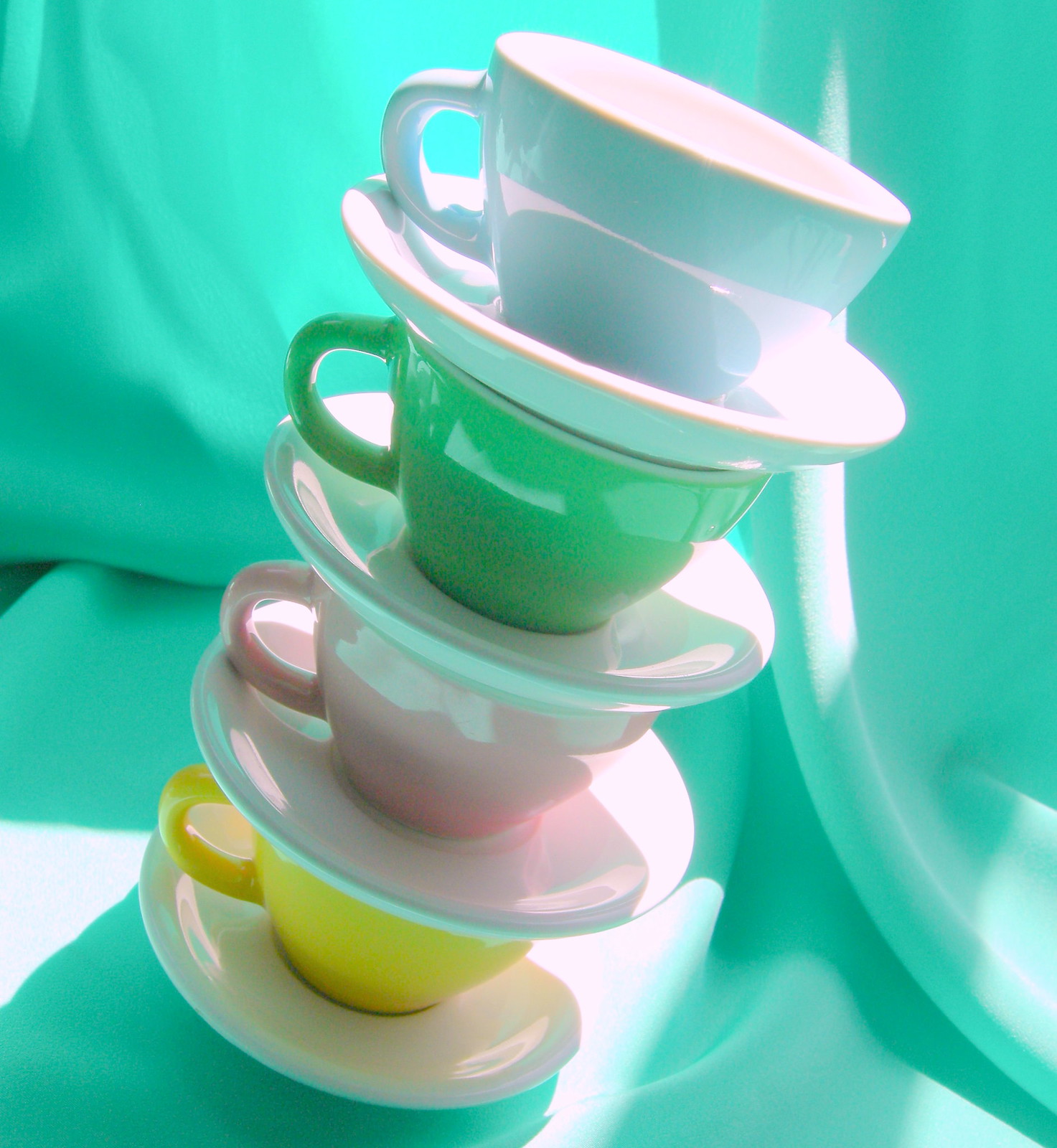The image captures a close-up photograph of a precarious stack of four teacups, each resting on a matching saucer, leaning slightly to the right at approximately a 45-degree angle. The backdrop is a draped, pale green sheet with some white spots, illuminated by sunlight peeking through, casting shadows and reflections on the teacups and saucers. Starting from the bottom, the cups and saucers follow this sequence: a white saucer with a yellow cup, a white saucer with a pink cup, a white saucer with a green cup, and finally, a white saucer with a white cup featuring a gold rim. Each teacup has a small handle positioned on the left side, and the sunlight enhances the ceramic glaze, making the teacups glimmer. The entire assemblage leans engagingly against the textured, softly-lit background.